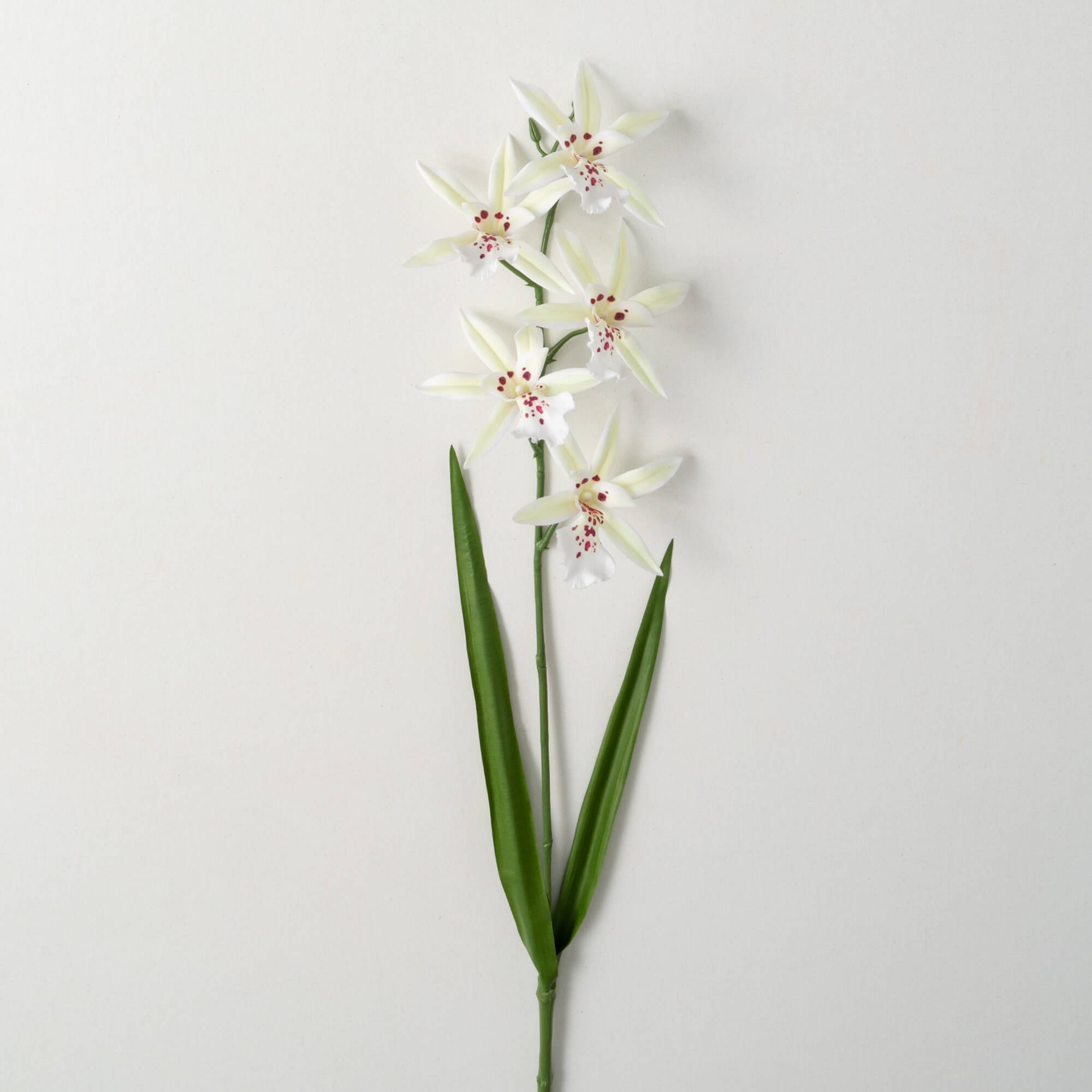This is a professional photo of a single green stem of flowers, likely artificial but with realistic detail, lying against a white or light gray surface. The image, taken from a vertical top-down perspective, features five star orchid-like flowers spaced along the main stem, each extending from its own short green offshoot. The flowers are predominantly white with six petals each, adorned towards the center with purple (alternatively described as red) polka dots. Additionally, the stem includes two long, narrow, pointed leaves that are positioned upwards near the bottom. A notable detail is the presence of a green bud at the topmost flower, which has not yet opened. The composition and lighting suggest a professionally taken photograph, showcasing the intricate and delicate beauty of the flowers.